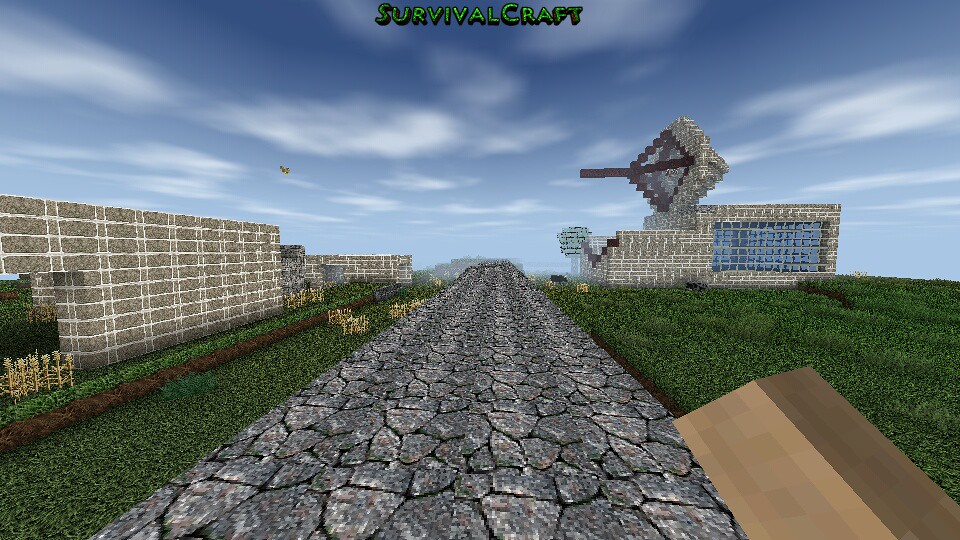The image is a screenshot from the video game SurvivalCraft, evident from the green text with a black outline at the top center of the screen. The overall aesthetic is pixelated and boxy, consistent with the game's graphical style. Dominating the center of the image is a gray cobblestone path that extends into the distance, leading towards the horizon. This path is flanked by lush green grass on either side. On the left, there are various buildings, some of which appear to be growing golden crops, possibly wheat, with stacks that resemble bales of hay. A gray brick wall with a hollow, square-like opening is also visible in this area. To the right, in the bottom corner, the hand of a Minecraft-like character can be seen, and nearby, there's a building with large blue glass windows, possibly made of bricks. This building is unique due to a gray, diamond-shaped object with a dark gray line sticking out from its top, somewhat reminiscent of a stone satellite. The sky above is a rich blue, gradually lightening towards the horizon, dotted with white, wispy clouds. Further along the road, another brick structure is visible, featuring glass elements and a tree at the far end.